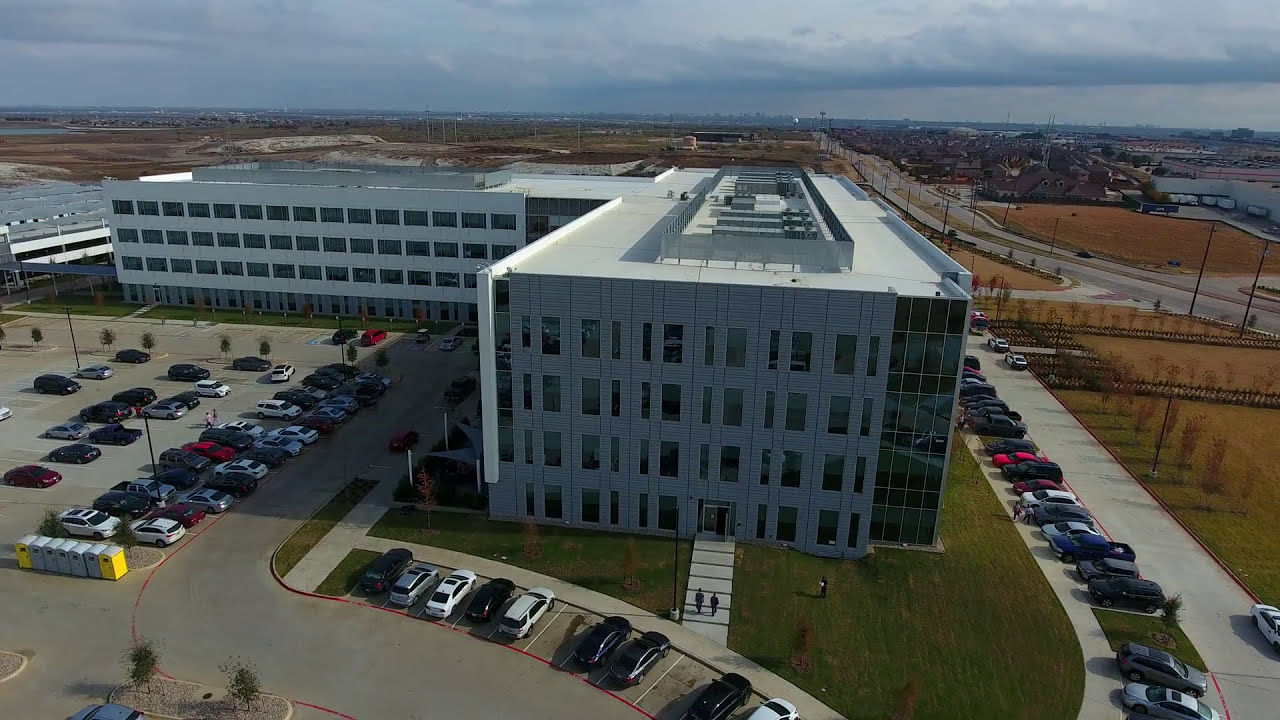An aerial view showcases a large, four-story L-shaped building surrounded by multiple parking areas. The building is constructed from white and light gray concrete, with a flat roof featuring a steel silver barrier and potential air conditioning units. The structure is adorned with numerous tall, narrow windows, and a prominent glass paneling running all four stories on the right side. 

To the left, within the L's interior, lies a parking structure made of the same white concrete, filled with cars and a row of port-a-potties. Additional parking extends to the front and right side of the building, connected by light gray asphalt driveways. A walkway with black lines leads up to the main entrance from a curving sidewalk, flanked by a well-kept green lawn. 

Towards the bottom right corner of the image, a narrow driveway appears, with a white car and several others parked beside it. Scattered decorative trees and tall lampposts, potentially equipped with cameras, enhance the parking areas. In the distance, a desert-like landscape gives way to a city's skyline under a dark, hazy sky filled with low, gray rain clouds.